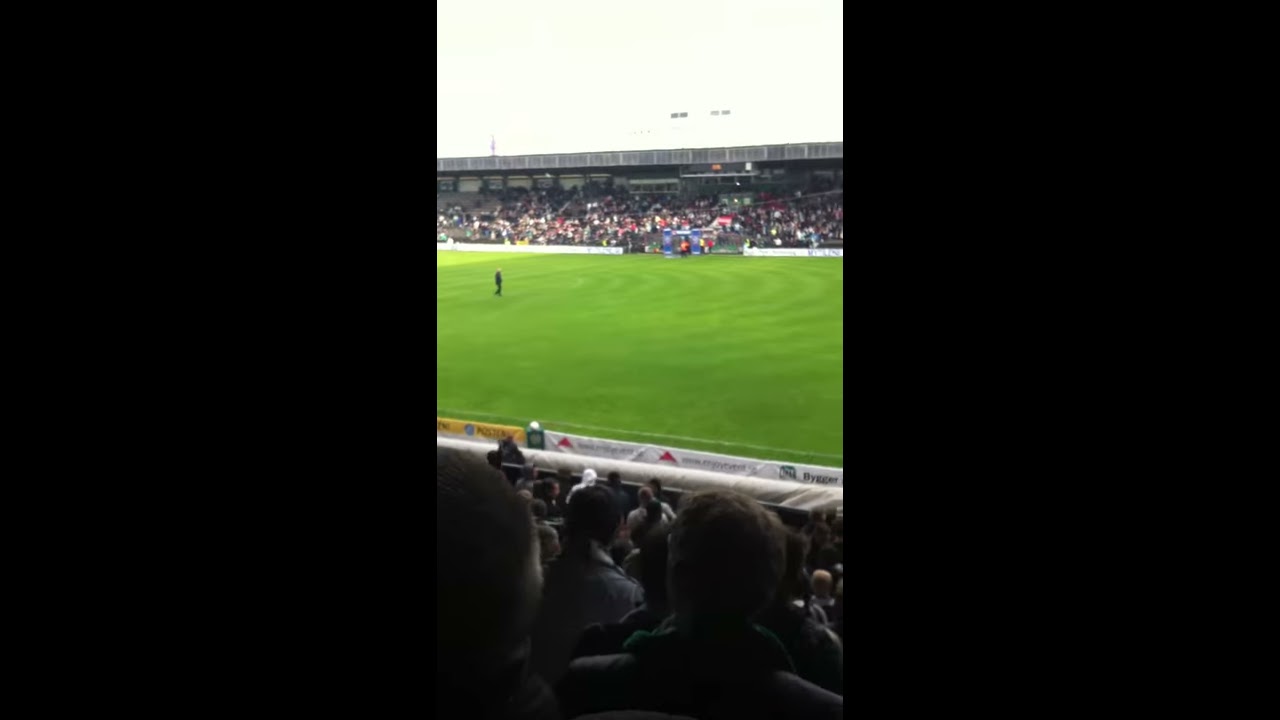The image depicts an outdoor stadium during a daytime event, crowded with spectators filling the stands both in the foreground and background. The photo is captured from a midpoint vantage in the stands. In the center, there's a large, green, unmarked field, indicative of it being either a soccer or some other type of sports field, but no clear lines or markings identify the specific sport. One person, possibly a coach or another official, dressed in black, is seen walking alone on the field in the distance. Although the sky appears gray, indicative of typical overcast weather, no lights are on, implying it's still daylight. In terms of color, the image shows a palette including black, gray, green, yellow, blue, red, and tan. There is no text visible anywhere in the image.